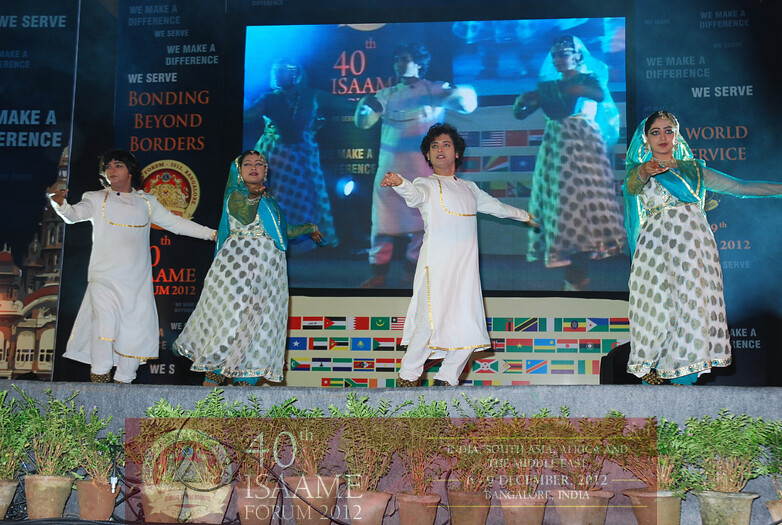The image depicts a vibrant cultural performance with four individuals, two men and two women, on a gray stage adorned with potted green plants lined up front. The performers appear to be of Arabic or Indian descent, aged between 35 to 40 years. The men, positioned on the left and right sides of the stage, are dressed in elegant white gowns with matching pants, their curly black hair completing their traditional look. The women, wearing sophisticated white dresses adorned with silver polka dots, accessorized with blue scarves and veils, and embellished with gold jewelry and heavy makeup, stand between them.

In the background, a large screen magnifies their image, accompanied by inspirational slogans such as "We Serve," "Bonding Beyond Borders," and "We Make a Difference," alongside a visible Bangladesh logo. Multiple flags from various countries also embellish the setting, adding to the international essence of the event. The screen and stage display text indicating "40th ISAE Forum 2012." The scene is well-lit by natural light, enhancing the clarity and prominence of the performers and their intricate, culturally significant attire.